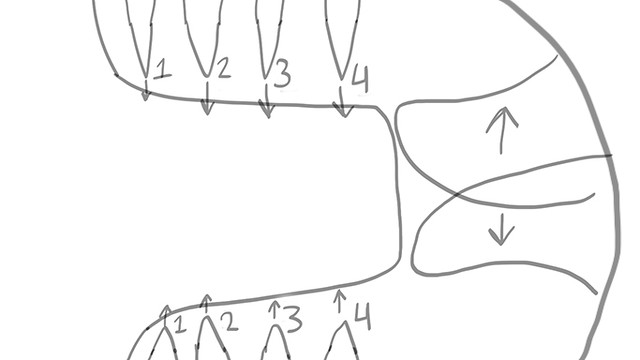This color diagram, rendered in a brown marker, features a prominent curved line starting from the left-hand corner, extending to the right, plunging steeply downward, and then curving back to the left. At the top of this line, 'V' shapes labeled with numbers 1 through 4, marked with arrows, direct along the line's path. Following the steep descent, the inverted 'V' shapes reappear, also numbered 4 through 1 in reverse order, with '1' proximal to the edge. On the right side of the diagram, two overlapping circles are connected by a solid brown line. Each circle has a brown arrow; one points upward from the top circle while the other points downward from the bottom circle, indicating directions along the outer edges of the circles.